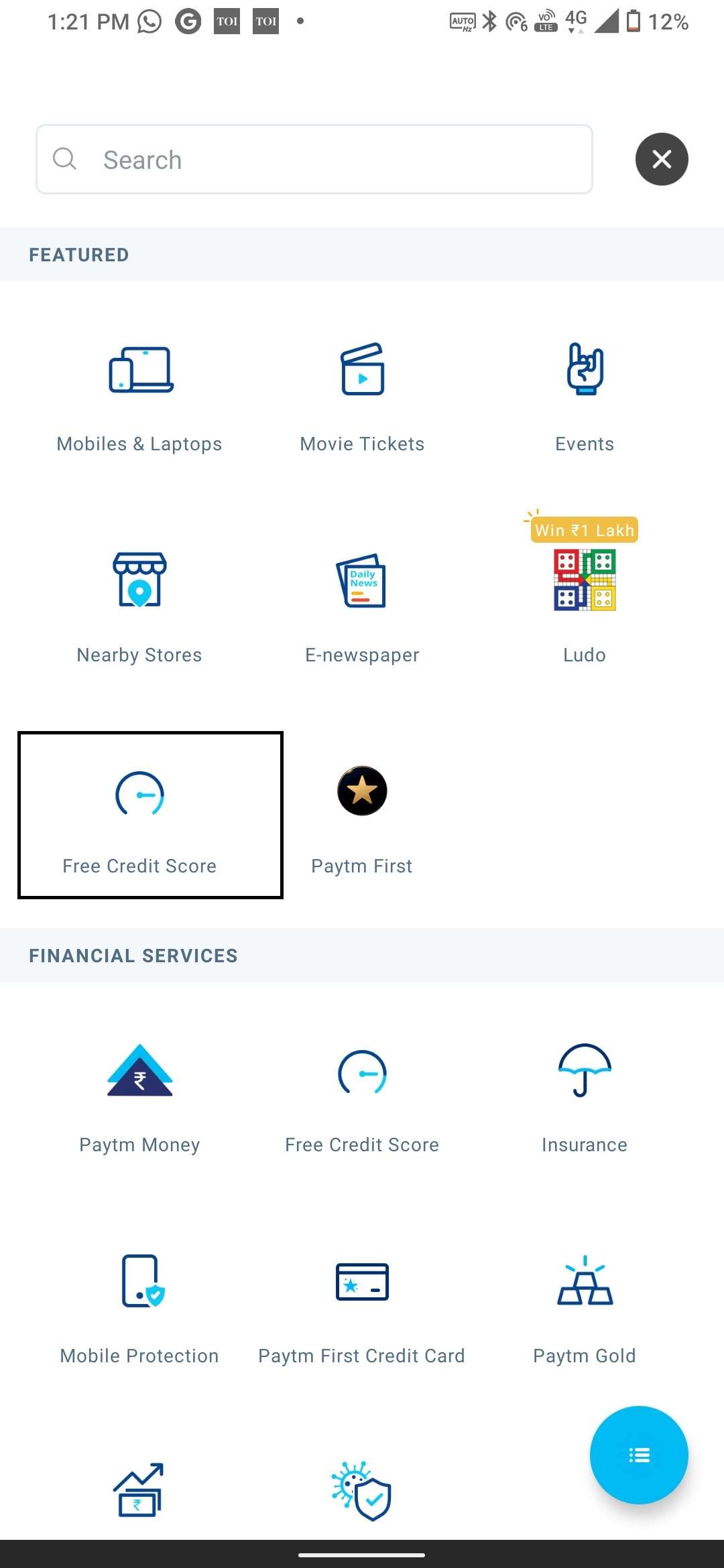The image appears to depict an app interface dominated by shades of blue, white, and black. The interface highlights various financial services, including features such as "Free Credit Score," insurance options, and payment solutions. Additionally, it offers ancillary services like e-newspapers, mobile and laptop services, movie tickets, and event bookings. The prominent use of blue suggests it is the brand's primary color. Notably, a multicolored logo spells out "Ludo," the only element with varied colors. The interface seems to be a prototype, as evidenced by two main sections labeled "Featured" and "Financial Services," both displaying the same options, particularly the "Free Credit Score." The "Free Credit Score" feature is encased in a square, indicating it is currently selected. Hence, the image likely showcases an app, possibly a credit card application that integrates various financial and lifestyle services.